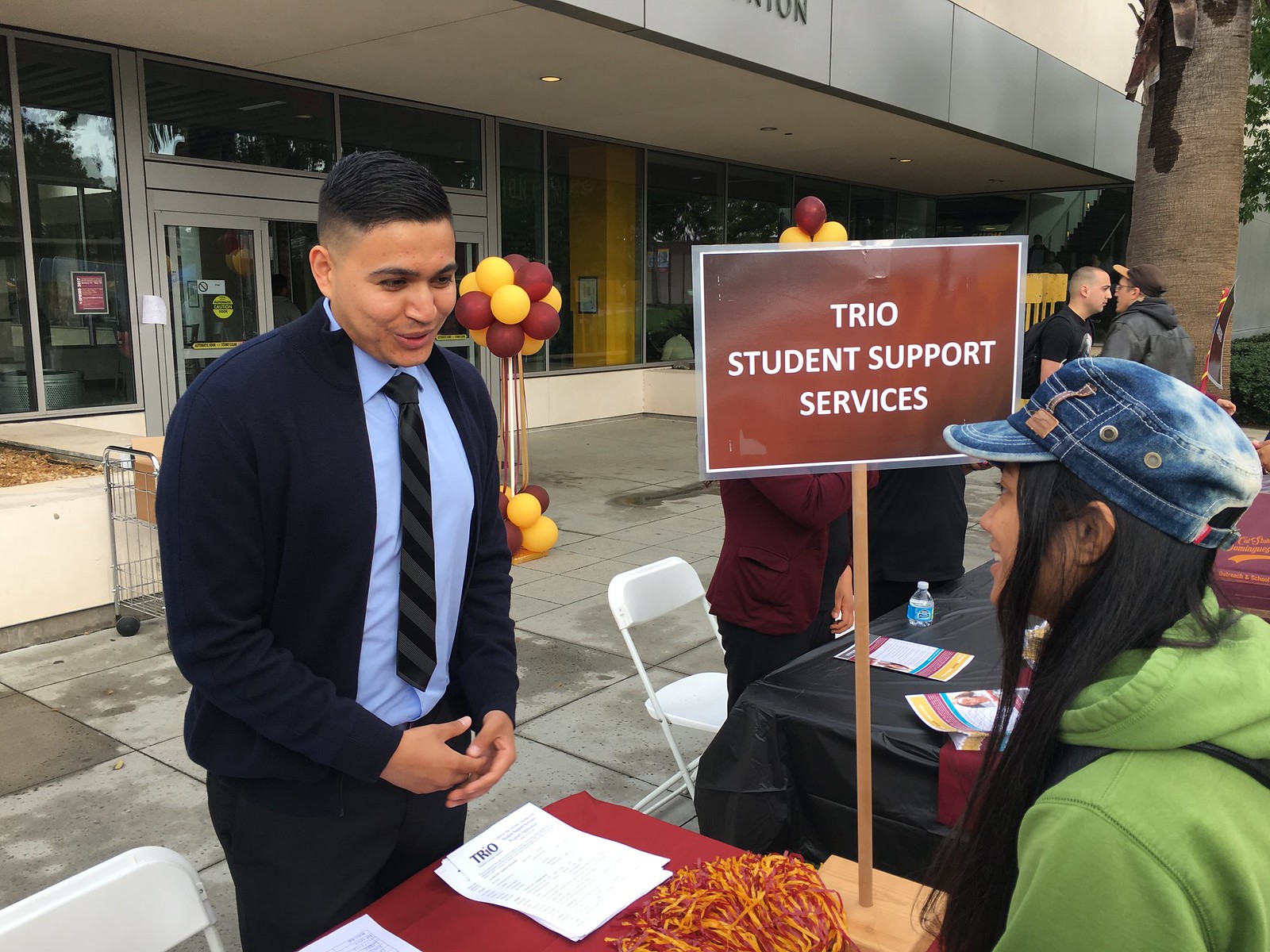The image captures an outdoor event, likely representing an organized activity, featuring multiple tables with various offerings. Central to the scene is a table draped in a maroon tablecloth, with a brown and orange sign atop a wooden post reading "Trio Student Support Services" in white letters. Positioned behind this table is a young Latino man in his 20s, attired in a blue dress shirt, a dark blue cardigan, a grey and black striped tie, and dark pants. He is engaged in conversation with a woman, seen from her profile, who appears to be Black, with long straight black hair, a blue denim cap, and a green hoodie. Papers bearing the Trio branding are spread on the table, along with what seems to be a bowl of spaghetti. To the right of the main pair stands a white folding chair. The scene is framed by a building entrance featuring glass windows and hanging gold and maroon balloons. In the upper right corner, additional tables host more interactions; one table has a black tablecloth with two people conversing, and nearby stands a tree trunk. The background reveals further tables and two men in discussion, suggesting an active and bustling event environment.